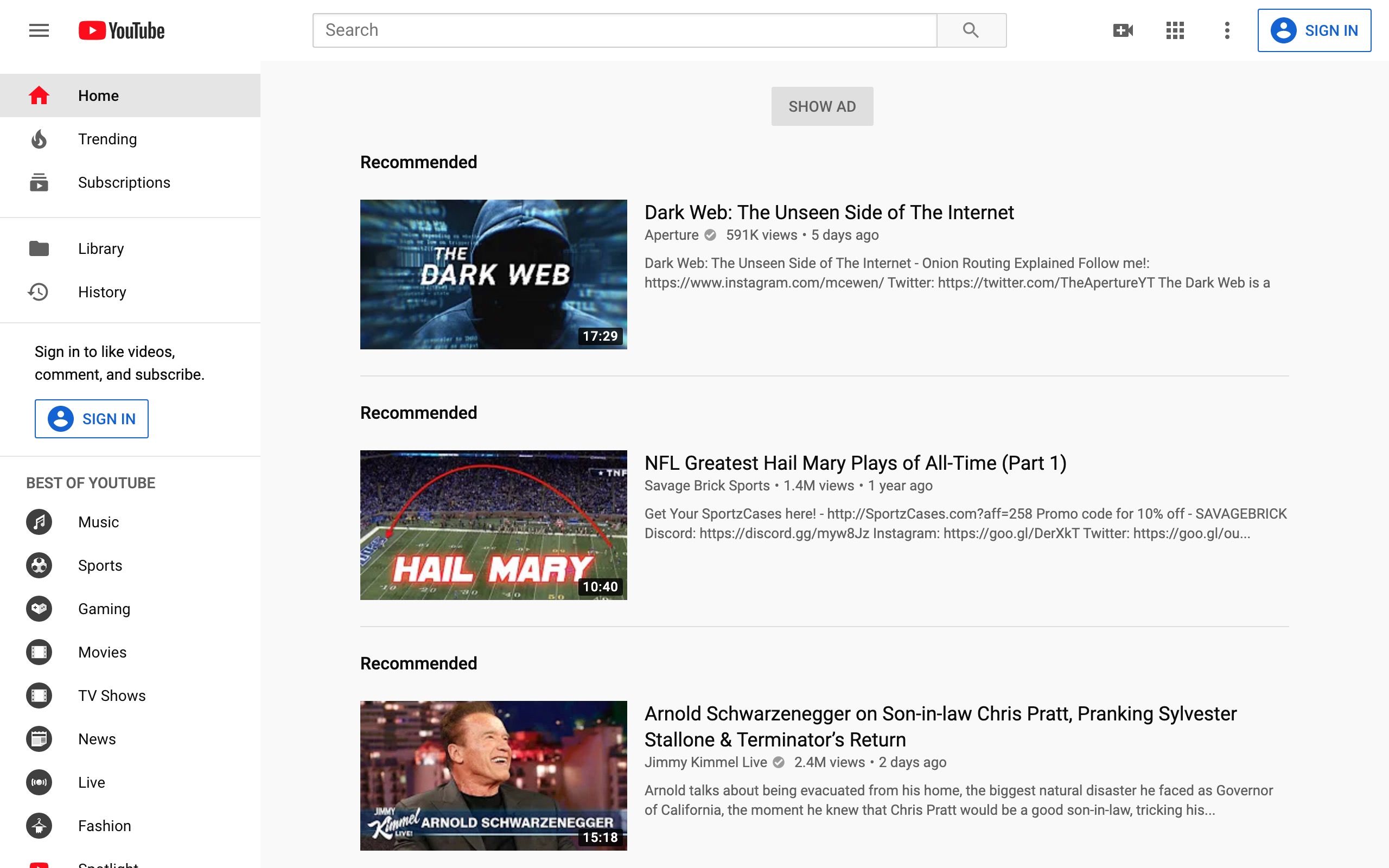A screenshot taken from a YouTube webpage displays three recommended videos for the user. On the left sidebar, there are multiple icons representing various sections of the website. At the top, the "Home" icon features a red house, indicating the user has selected this section, as the word "Home" is written beside it in bold. Below, additional icons are labeled as "Trending" and "Subscriptions." A faint gray line divides these from the next section, which includes "Library" and "History."

Another faint gray line beneath these sections suggests a prompt for users to sign in, featuring the text: "Sign in to like videos, comment, and subscribe," accompanied by a sign-in button showing a blue circle with a white silhouette of a person. Under the category "Best of YouTube," several icons are listed sequentially: Music, Sports, Gaming, Movies, TV Shows, News, Live, and Fashion, though the list cuts off before the final option.

The recommended videos showcased in the center of the screen are as follows:
1. "Dark Web: The Unseen Side of the Internet."
2. "NFL's Greatest Hail Mary Plays of All Time - Part One."
3. "Arnold Schwarzenegger on Son-in-Law Chris Pratt Pranking Sylvester Stallone and the Terminator's Return."